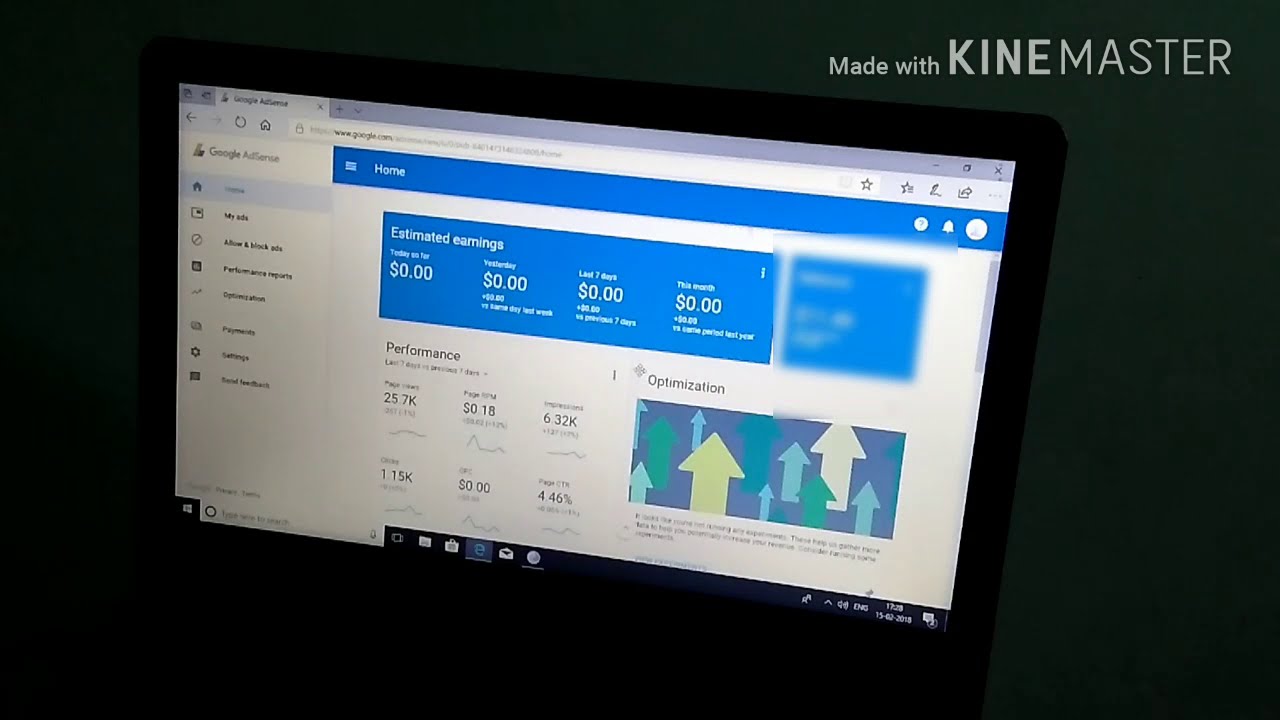The image presents a diagonally angled laptop screen against a dark gray background, featuring a website interface likely from an investment platform. In the upper right corner, in light gray letters, the watermark reads "Made With KineMaster." The main webpage display has a predominantly white background with black, blue, and light gray accents. At the top, the word "Home" is visible, followed by a prominent blue box labeled "Estimated Earnings," which lists values as zeros across four columns. Below, various performance metrics are displayed, including figures like 25.7K and 4.46%, though their exact indicators are illegible. On the bottom right, vivid arrows in yellow, green, and turquoise point upwards, signifying optimization features. The left sidebar contains various navigation options. The entire image is bordered in green, adding a frame to the composition.